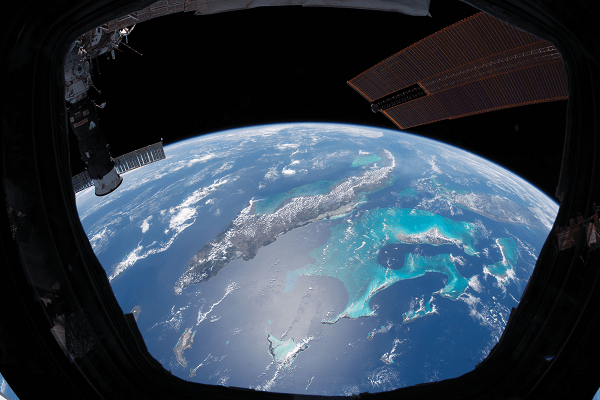The photograph, possibly computer-generated, showcases a stunning view from within a space capsule, satellite, or spaceship, orbiting high above Earth. The rectangular image, approximately four inches wide and three inches high, captures the curved arc of the Earth near the top, displaying its beautiful blue oceans and swirling white and gray cloud formations. From the window's perspective, you can see Earth's atmospheric layers with some areas of turquoise blue, hinting at lakes or oceanic regions.

Surrounding the visible section of the window is a dark metal framework, casting shadows that obscure certain details, contributing to the dramatic contrast against the bright planet. On the upper left, there is a mention of part of the International Space Station, while the upper right corner features a distinct five-sided object, possibly a visor or solar panel. Additionally, there's a wing of a satellite, characterized by a striated, brownish-red color, adding depth to the scene. The lower left includes another unclear object, potentially a microphone or camera. Overall, the photograph captures a mesmerizing glimpse of Earth and the technology that keeps us connected with space.